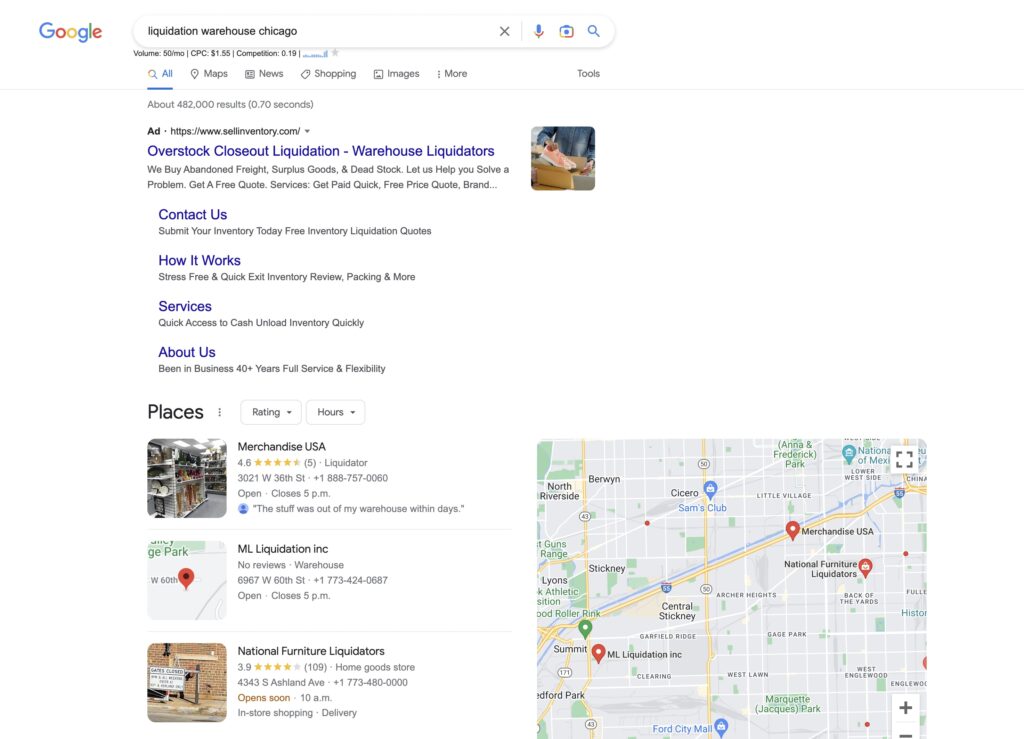The image shows a Google search results page for "liquidation warehouse in Chicago." At the top, the search field displays the query, accompanied by familiar icons such as the close button "X," microphone, camera, and magnifying glass. The Google logo is visibly positioned on the left, with navigation tabs including "All," "Maps," "News," "Shopping," "Images," "More," and "Tools."

The search yields approximately 482,000 results, starting with advertisements for companies like Overstock, Closeout Liquidation, Warehouse Liquidators, and others promoting services such as purchasing abandoned freight, surplus goods, and dead stock, with offers for free quotes and fast payment.

An illustrative thumbnail on the right shows a person extracting a pair of pink shoes from a box, with additional links below for "Contact Us," "How it Works," "Services," and "About Us."

The organic search results highlight various liquidation businesses. First is Merchandise USA, rated 4.6 out of 5 stars from five reviews, listed as a liquidator, complete with address, phone number, and business hours (currently open, closing at 5 p.m.). An interior shot of the store is provided.

Next is ML Liquidators Inc., which has no reviews or images, only a screenshot from Google Maps.

Following that, National Furniture Liquidators is mentioned, featuring a peculiar sign in front of a brick wall with a rating of 3.9 stars from 109 reviews, categorized as a home goods store.

On the right of the search results page, there's a small inset map displaying the locations of these businesses, provided by Google Maps.